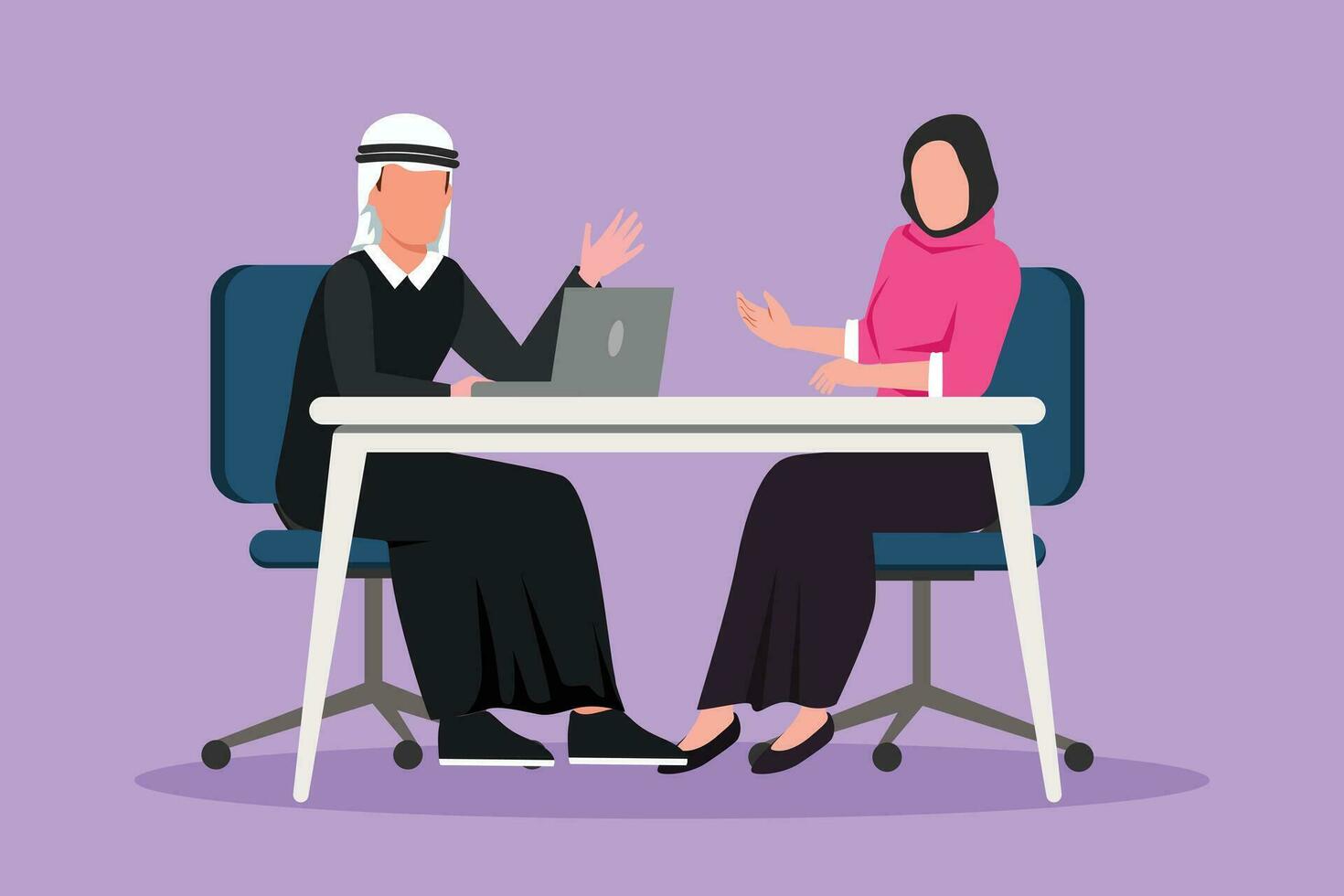This detailed illustration, possibly a computer rendering, portrays two individuals engaged in a discussion while seated at a white or gray table with two legs. The setting includes two aqua blue rolling chairs with wheels. The man on the left is distinguished by his white turban with a double black headband, traditional black robe, and black and white shoes. He is attentively working on an open gray laptop in front of him. The woman on the right, wearing a black headdress that reveals only her eyes, is dressed in a pink sweater over a rolled-up white long-sleeve shirt, paired with a black skirt and matching shoes. She seems to be gesturing towards the man as they converse. The overall background includes hints of purple, adding depth to the scene.